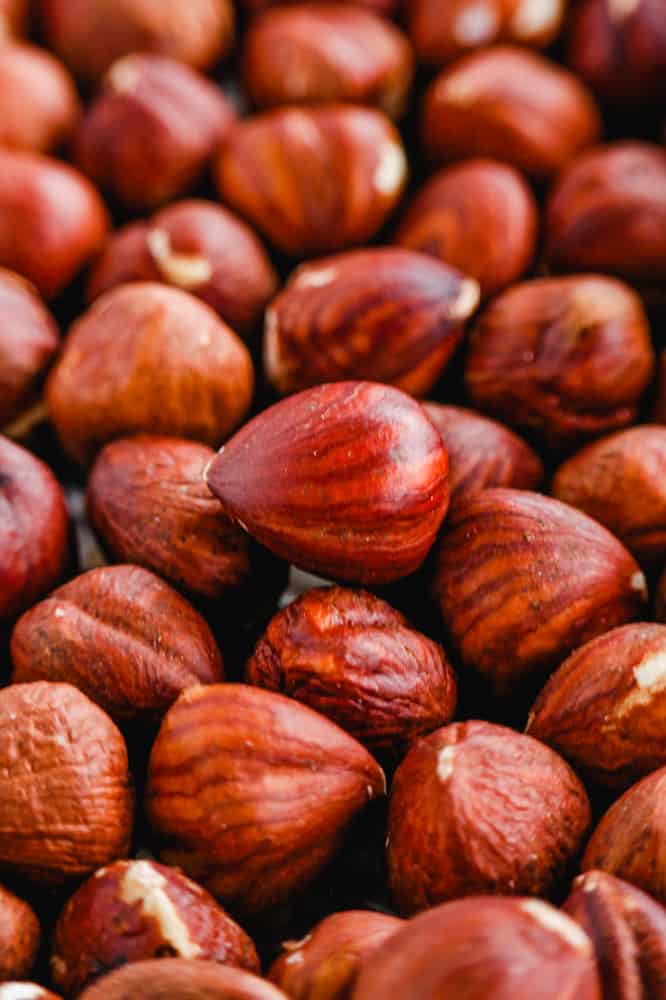This close-up image features an array of approximately 30 shiny, reddish-brown shelled hazelnuts with distinct maroon and tan stripes. The nuts, almond-shaped with a round bottom tapering to a teardrop point, are arranged in a somewhat scattered manner, layered atop one another on a dark, likely black surface which could be a table or cloth. The image is well-lit from above or possibly outdoors, with the top third of the photograph blurrier than the crisp, detailed foreground. A particularly large hazelnut sits prominently in the center, drawing immediate focus amidst the multitude of similar nuts dotting the scene.